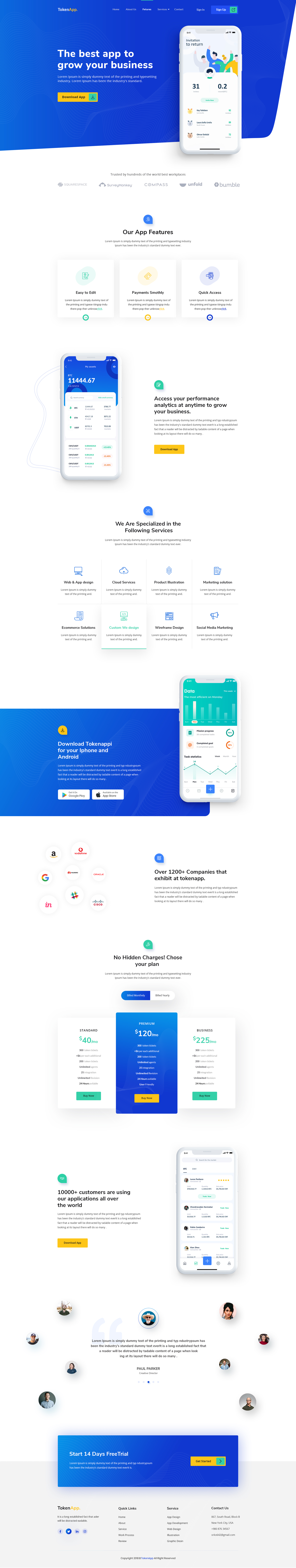The image is a detailed vertical screenshot of a business support application.

At the very top is an advertising banner with the slogan "The Best App to Grow Your Business" in bold white text, accompanied by additional text and a gold banner.

Adjacent to this is a small thumbnail image that reflects part of the larger screenshot. Below the banner are three main sections with dark text delineating the features offered by the app. These feature descriptions are followed by eight selectable subcategories.

Further down, a wide blue banner with white text dominates the screen, featuring two white text fields accompanied by small icons. Next to this banner is an image displaying a graph with green elements on a white background.

Proceeding downward, a central section highlights three options, with the middle one selected and highlighted in blue, while the other two are in white with small green action buttons beneath them.

Continuing further, there is another section containing a small paragraph of dark text with a bold headline and a gold action button beneath it. Adjacent to this is an image showing various selectable options arranged in a vertical column.

Towards the bottom of the screen, nine differently angled icons are displayed around a central body of text. Below this arrangement is a blue section with white text and a gold action bar.

Finally, at the very bottom, there are four columns of information presented in black text against a white background, completing the detailed layout of the app's screenshot.